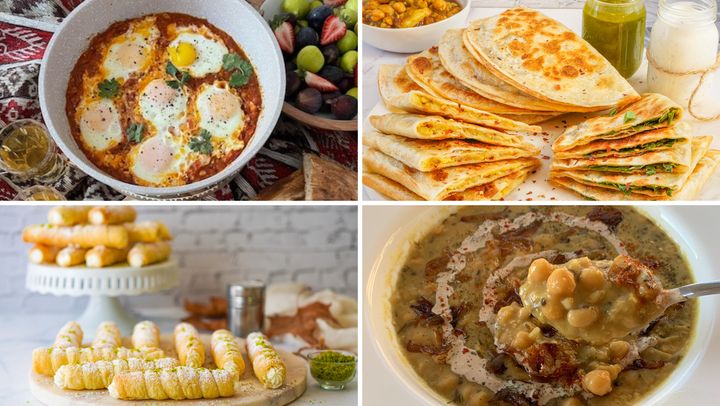The image presents a 2x2 grid of four food photographs, each bordered by thin white lines. In the top left quadrant, a white bowl brims with a tomato paste broth, garnished with several boiled eggs, possibly six, and a touch of green herbs. Adjacent to this, the top right quadrant features a white plate stacked with beautifully browned quesadillas, accompanied by two mason jars containing green juice and milk. The bottom left quadrant displays an array of cream-filled yellowish pastries, akin to cannolis, arranged on a brown oval cutting board with additional pastries on a cake stand in the background and a small clear container of green dusting. Finally, the bottom right quadrant shows a hearty bowl of brownish curry or stew with visible white beans and yellowish kernels, possibly resembling dal, with a silver spoon's handle peeking from the right. All these dishes rest on a tablecloth patterned in red, black, and white, giving a rustic charm to the vibrant spread.